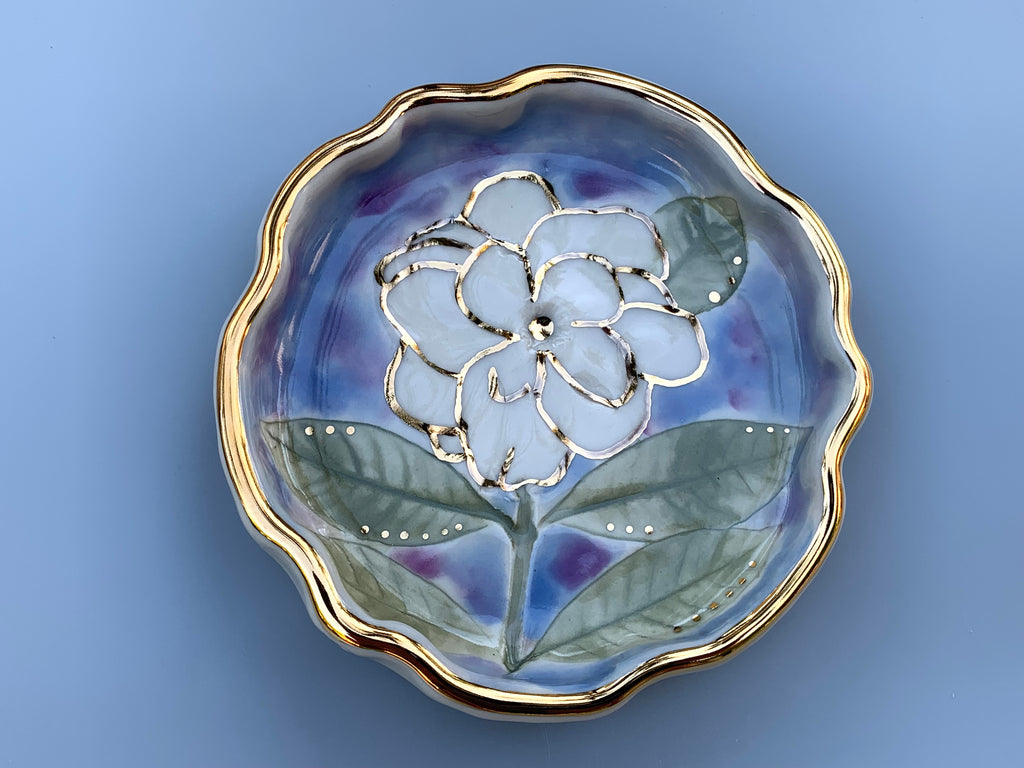This photograph captures a detailed top-down view of a small, curvy-shaped ceramic dish sitting on a light blue, possibly periwinkle, surface. The dish, which has a handmade appeal due to its wavy and imperfectly round edges, features a gold accent along its rim. Inside the shallow bowl, there is a beautifully crafted white flower with green stems and leaves. The petals are outlined in silver, as are the dots accenting the edges of the leaves. The background within the dish exhibits a tie-dye pattern of light blue blended with hints of purple, complementing the periwinkle surface the dish sits upon.